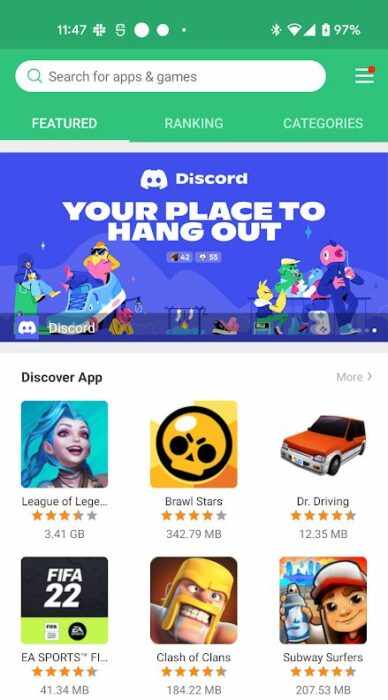This is a detailed smartphone screenshot featuring an app store interface. At the top, the device's time is displayed as 11:47 AM, accompanied by an array of status icons: a cross symbol, an S shape or a dollar sign, and three white circles that decrease in size from left to right. On the far right, familiar status icons are present: Bluetooth, Wi-Fi, cellular signal, and a battery icon indicating a 97% charge.

Just below the status bar, there is a search bar awaiting user input. Immediately beneath the search bar, an advertisement for the app "Discord" appears, promoting it as "Your place to hang out." The ad creatively depicts various whimsical creatures resembling fish, dogs, and other fantastical beings, all engaging in a festive outdoor gathering, suggestive of a campout or picnic.

Further down, a section labeled "Discover App" introduces a selection of app icons. This area is neatly organized into two horizontal rows, each containing three app icons. The first row showcases "League of Legends," "Brawl Stars," and "Doctor Driving," while the second row features "EA Sports," "Clash of Clans," and "Subway Surfers." Each app icon is clearly presented, inviting the user to explore popular gaming options.